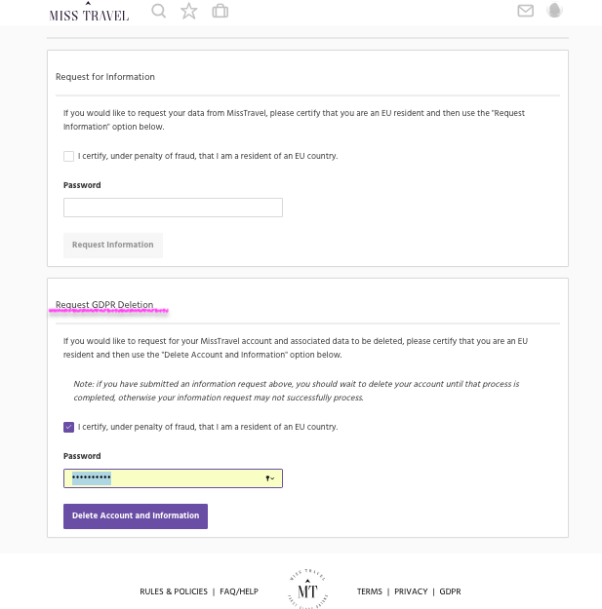Screenshot of a Personal Information Page on the Mistravel Website:

At the top left corner of the webpage, the bold letters "Mistravel" stand out against a white border. To the right of the name, there are five icons: a magnifying glass, a star, a suitcase, an envelope, and an icon resembling a palm.

The body of the page has a gray background, with a prominent white box positioned at the top. This box is titled "Request for Information" in small black letters. Below the title, there's a detailed explanation on how to initiate the request process. An option to certify EU residency is provided as a checkbox within this section. At the bottom of this box, the word "Password" appears, followed by a grayed-out button labeled "Request Information" on the bottom left.

Lower down the page, a second white box is present. It is titled "Request GDPR Deletion," emphasized with an underlined pink line. This section contains similar certifications and descriptions as the first box. At the bottom left of this box, a button labeled "Delete Account and Information" stands out in a vibrant purple color.